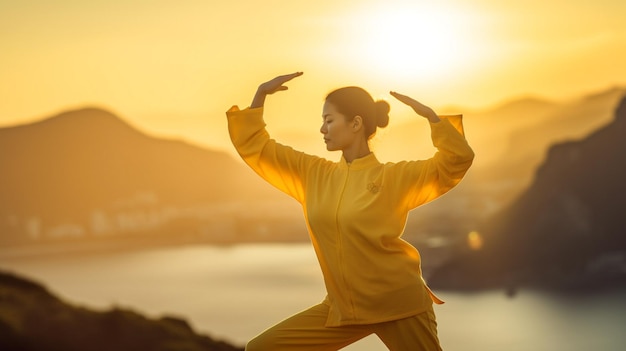In the image, an Asian woman is seen exercising outdoors against a vibrant, yellow-tinted backdrop. She is wearing a long-sleeved, yellow zip-up tunic-style top with matching yellow pants. Her dark hair is tied up in a bun on the back of her head, and she gazes seriously towards the left side of the image. The photograph cuts off at her knees, showing her right leg extended with the right knee bent, while her left leg is slightly behind her. Her arms are raised in a curved, crab-like pose, with elbows bent and fingers pointed above her head. 

The background features a scenic view of a lake flanked by mountains on both sides, creating a serene and picturesque setting. To the right above her, the sun shines brightly, casting a white glow in the yellow sky and sending a sun ray past her right shoulder. The overall ambient yellow hue suggests either a filter applied to the image or soft morning or evening light, enhancing the tranquil atmosphere of the scene.